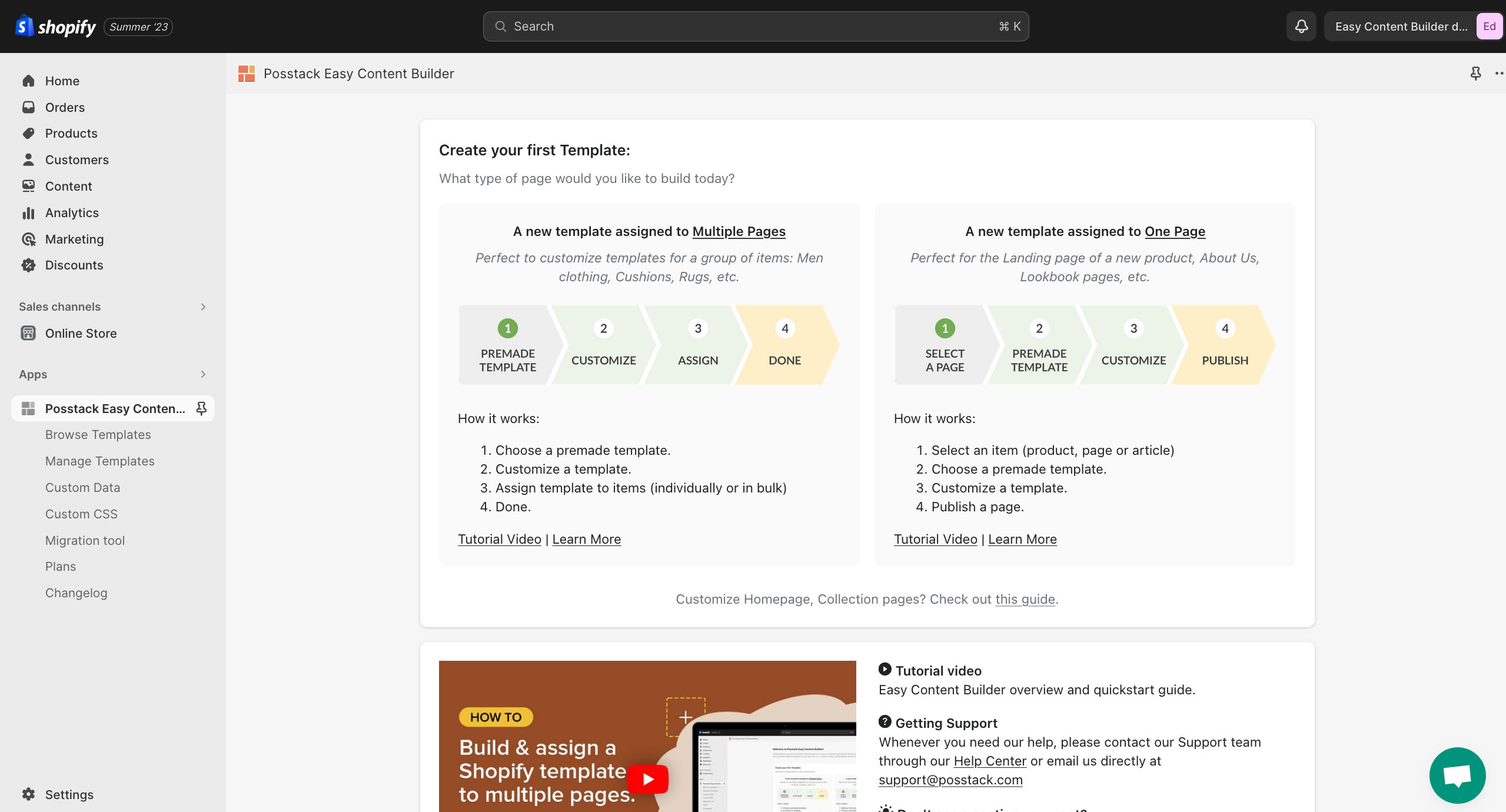The image is a screenshot of a web page displayed within the Shopify platform. At the top of the screen, the Shopify logo is prominently visible. The main content features a blue bag illustration. On the left side of the screen, there is a vertical, gray sidebar with various navigational sections including “Home,” “Orders,” “Products,” “Customers,” and more, which extend further down.

In the center of the page, there is a section titled "Post-Stack Easy Content Builder." Below this heading, instructions for creating a template are displayed, which include the phrase “Create your first template.” This section is organized with arrows indicating steps in a process: from the first step to the fourth, illustrating a clear workflow.

The instructions cover how to create a new template, including options for assigning a single template to one page or to multiple pages. Towards the bottom of the screen, a partially visible section provides further details on "How to build and assign a Shopify template to multiple pages," complete with bullet-points and step-by-step instructions in black text. In the lower right-hand corner of the display, there is a green help button and a speech button, providing additional support options.